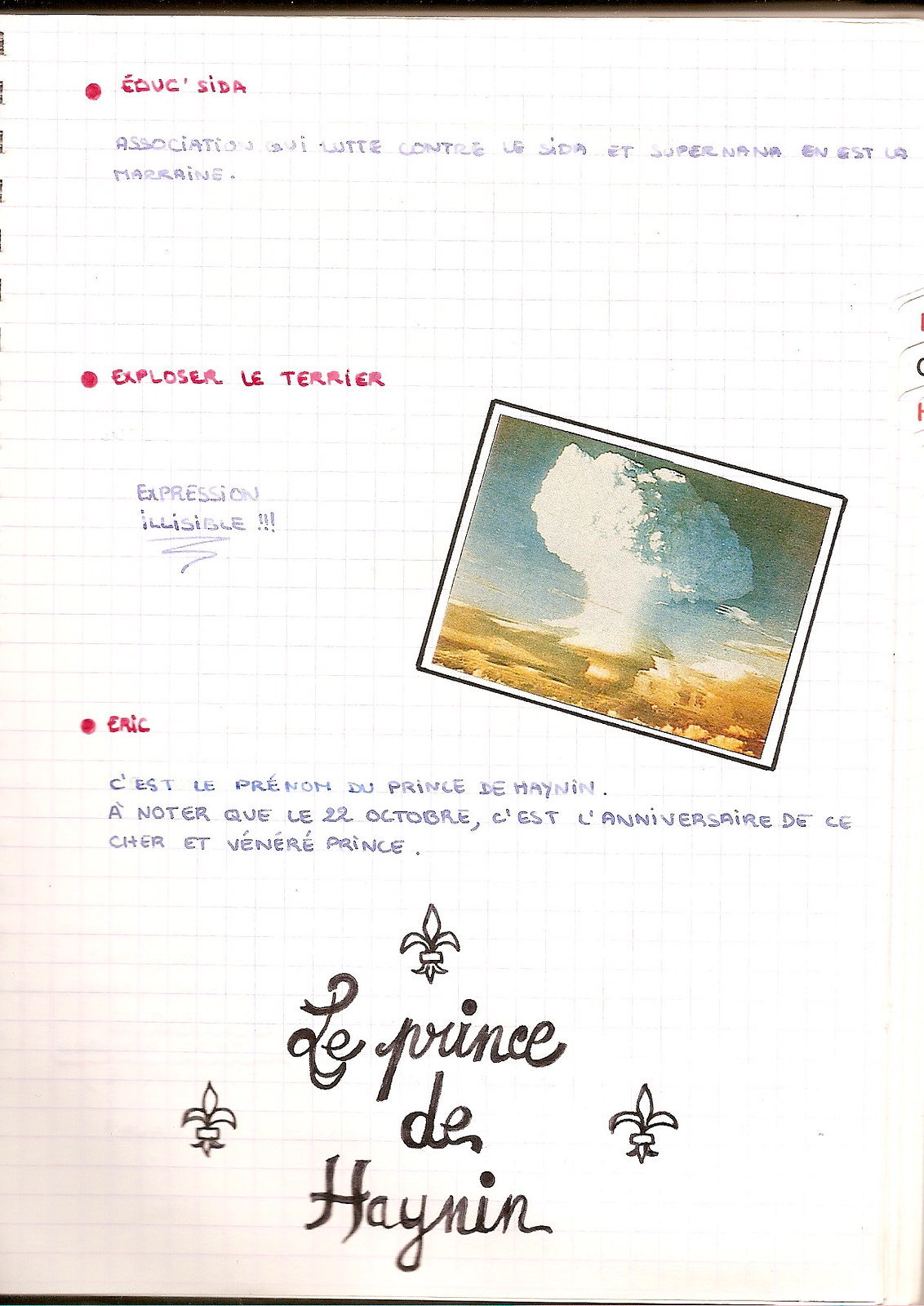The image is a colored photograph of a notebook page with grid lines, resembling graph paper. The notebook appears to be photocopied, with rows of vertical and horizontal lines. At the top, the text is written in red ink, featuring the letters "E-O-U-C-S-I-D-A," possibly French. The next red line legibly reads, "E-X-P-L-O-S-E-R L-E-T-E-R-R-I-E-R," followed by the word "Expression" and another illegible word. In the center of the page, there is a tilted color photograph of a large explosion creating a mushroom cloud, set against an orange, dirt-filled terrain.

Beneath the photograph, in red ink, is the repetitive line "E-R-I-C E-R-I-C E-R-I-C." Below this in black ink, a French passage reads, "C'est le prénom du prince de Heinen. À noter que le 22 octobre, c'est l'anniversaire de sa chère et venerie prince." At the bottom of the page, in cursive script, it says, "le prince de Heinen," spelled "H-A-Y-N-I-N."